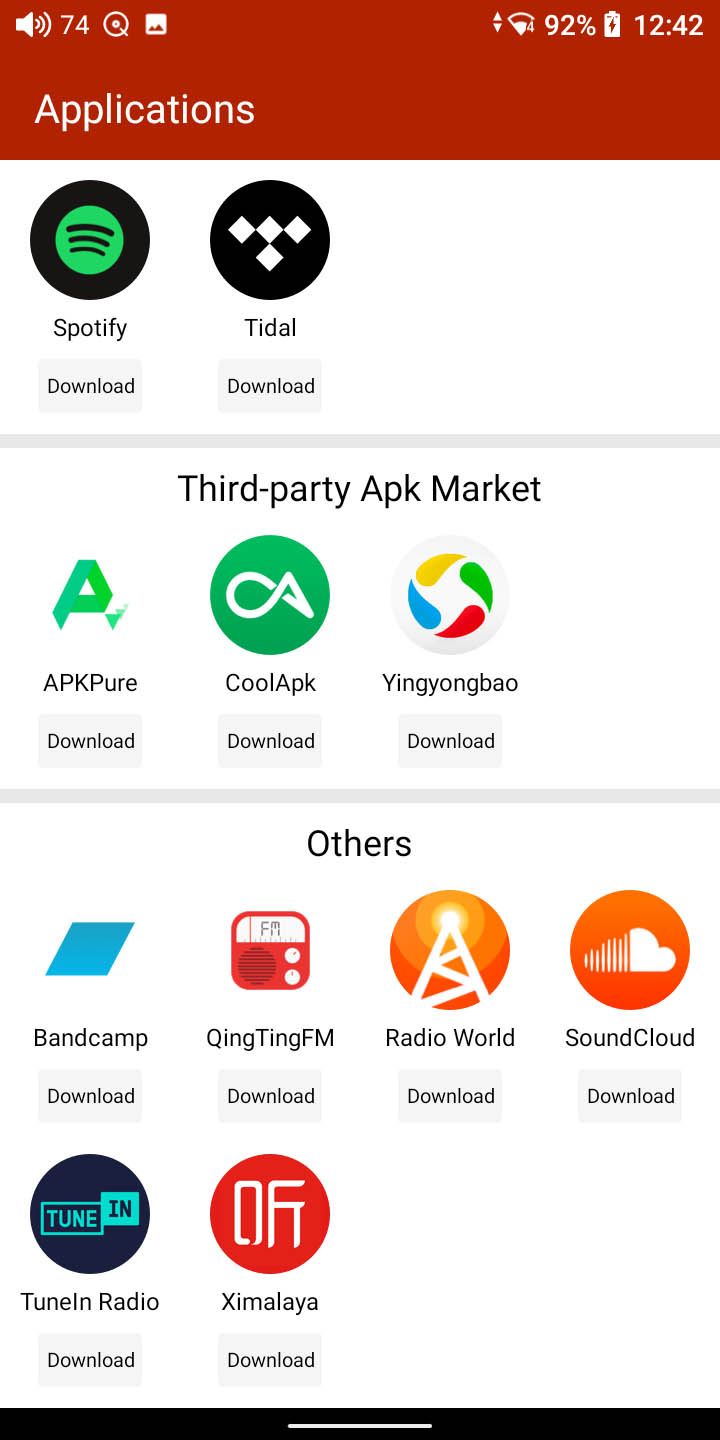The image displays an Android AI interface. At the top, there's a red box labeled "Applications" with white text beneath it. Below, the interface showcases two black circles featuring app icons: one with a green logo representing Spotify, and the other with a white four-diamond logo for Tidal. Both apps have a "Download" option underneath them.

A gray separator line follows, categorized as "Third-party APK Market." Listed here are APK options including APKPure, APKCool, and APKK Yin-Yang Bao. 
- **APKPure**: Denoted by a green circle with a white logo.
- **APKCool**: Also represented by a green circle with a unique white logo.
- **APKK Yin-Yang Bao**: Illustrated with water droplets in red, green, yellow, and blue, arranged in a ying-yang pattern.

Each option has a "Download" button below them.

Another gray line separates this section, labeled "Others." The listed apps in this section are Bandcamp, Qing Qing FM, Radio World, SoundCloud, TuneIn Radio, and Ximalaya.
- **Bandcamp**: Represented by a blue triangle.
- **Qing Qing FM**: Features an old-school red radio icon.
- **Radio World**: Depicted with an orange radio tower icon.
- **SoundCloud**: Shows a white cloud fragment within an orange circle.
- **TuneIn Radio**: Simply states "TuneIn" within a dark blue circle.
- **Ximalaya**: Displays white Chinese characters on a red circle background.

In the top-right corner of the interface, the time is displayed as 12:42.